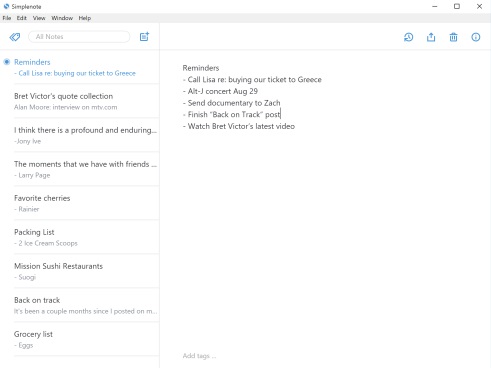The image showcases a note-taking application interface, prominently labeled "Simplenote" at the top, marked with a distinctive blue Earth icon. Below the title, a classic menu bar displays options such as File, Edit, View, Window, and Help, all in black font. Directly beneath this menu is a search bar designed for finding specific notes. An icon for creating a new note is visible, alongside additional icons for sharing or deleting notes.

The central section of the interface lists approximately eight different notes. The first note, titled "Reminders", is highlighted in blue, indicating it is currently selected. It contains a reminder to "Call Lisa" regarding the purchase of tickets to Greece (RE: buying our tickets to Greece). Other notes include:

- "Brett Victor's Quote Collection" featuring an "Alan Moore interview on MTV.com".
- An incomplete thought: "I think there is a profound and enduring," attributed to Janie Hugh.
- "The moments that we have with friends," with a reference to Larry Page.
- "Favorite cherries," noted as Rainier.
- "Packing list," which mentions "two ice cream scoops".
- "Mission Sushi Restaurants" with the mention of "Sugi" and a partial note stating, "Back on track. It's been a couple of months since I posted on my..."
- "Grocery list," beginning with "eggs".

Each note in the list appears as a preview, which upon selection, displays the entire content in the central reading pane of the application.